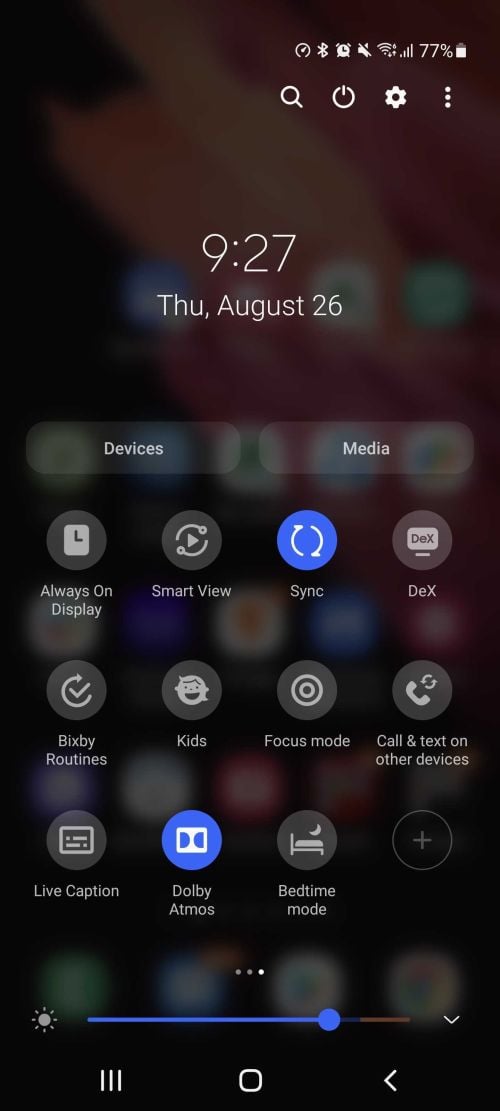Screenshot of a Phone Interface with Quick Settings Panel Displayed

In this detailed screenshot of a smartphone's interface, the time and date, "9:27 AM, Thursday, August 26th," are prominently displayed at the top. To the right of the time, several status icons are visible, including a battery charge indicator, an alarm clock icon, a magnifying glass, a power button, a gear icon, and a series of dots representing additional options.

Below the date, two transparent buttons labeled "Devices" and "Media" are presented. The main section of the screen showcases an array of quick setting icons organized in rows, each indicating different functionalities. 

1. Always On Display
2. Smart View
3. Sync (Highlighted in blue)
4. Dex (with 'DE' in capital letters)
5. Bixby Routines
6. Kids Mode
7. Focus Mode
8. Call and Text on Other Devices
9. Live Caption
10. Dolby Atmos (Highlighted in blue)
11. Bedtime Mode (Adjacent to a plus (+) icon)

Beneath these settings, three small dots suggest additional pages of quick settings. Further down, a brightness adjustment bar is visible, marked by a sun icon, with a blue slider positioned towards the right, indicating a higher brightness level.

At the bottom of the screen, three navigation icons are located:
1. Three vertical lines on the left
2. A roundish square in the center
3. An arrow pointing to the left on the right

The layout is clean and intuitive, providing quick access to essential settings and features.